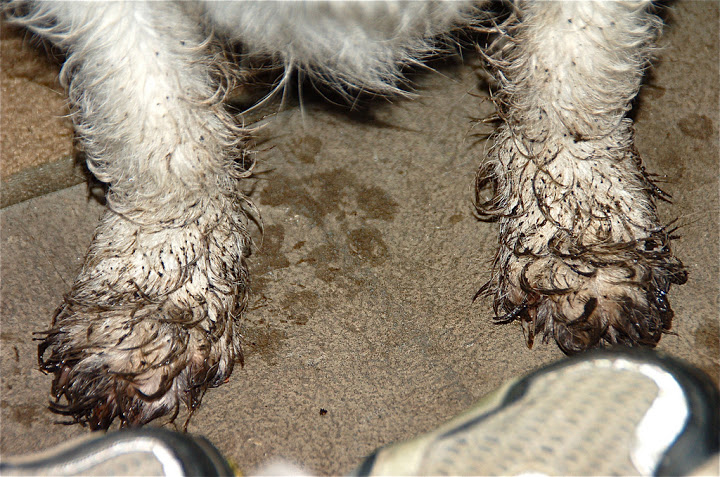This close-up image focuses on the muddy paws of an animal, likely a dog but possibly a cat, with white fur matted and dirty from mud. The animal's lower body and legs are partially visible, revealing patches of clean white fur amidst the grime. The animal is situated on a surface that appears to be a tan-colored rug, with part of its paws extending onto a floor that could be either tile or concrete. The wet paws have left muddy prints and water spots on the floor. In the foreground, there is an indeterminate object, possibly a shoe or glove, featuring reflective trim and black material. The scene vividly captures the mess created by the animal, emphasizing the stark contrast between the white fur and the dirt.